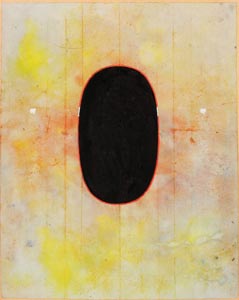This image depicts a modern art painting characterized by a predominantly off-white or light gray background with marbled textures. Yellow and orange splotches fill the upper left side and bottom of the image, interspersed with hints of red and occasional brown spots, particularly on the lower right. A central, vertically aligned black oval dominates the composition, surrounded by a thin red border with small white interruptions on the left and right sides. The painting also features vertical streaks in brownish-red hues, reminiscent of wall paneling, which align closely around the oval, adding structure to the abstract arrangement of colors and textures.